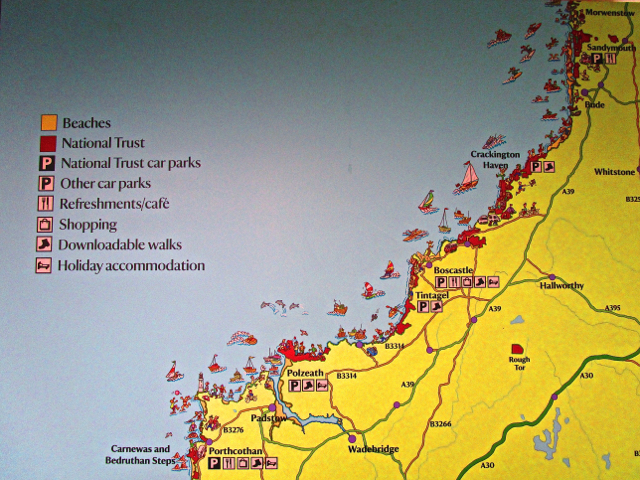The image depicts a detailed and colorful map of a coastal tourist area, characterized by a yellow landmass and a bluish-gray body of water. Major roadways are highlighted in green, while minor ones are marked in red. Key towns and cities such as Hallworthy, Boss Castle, Tintagel, Polsey, and Porthcothen are labeled, although some names are difficult to read.

The left side of the map contains a comprehensive legend with various icons: an orange square indicating beaches, a red square for National Trust sites, a black-on-white 'P' for other car parks, and a white-on-black 'P' for National Trust car parks. Additional icons include utensils for Refreshments/Cafes, a shopping bag for Shopping, a boot for Downloadable Walks, and a bed for Holiday Accommodations. The coast is tinted red, presumably marking National Trust areas, and the beaches are highlighted in orange.

The map is adorned with small, illustrative icons of boats, fish, and dolphins, as well as images of people vacationing, adding to the lively, tourist-friendly theme. The clarity and quality of the map facilitate easy navigation for visitors seeking to explore the area's attractions and amenities.